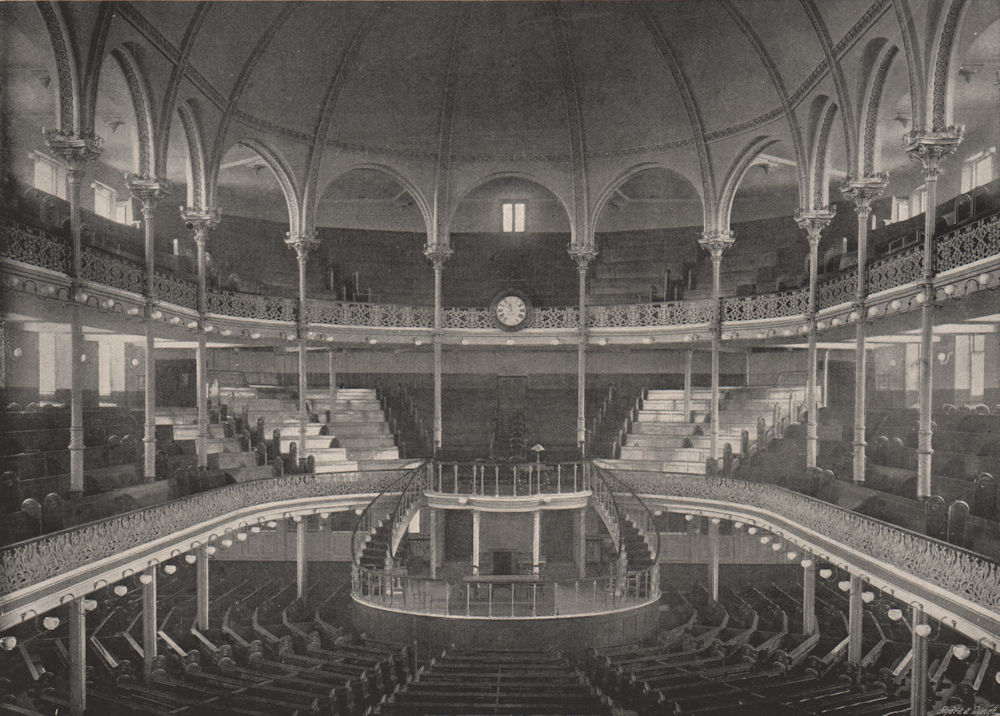This image captures the grand interior of an ornate theater or stadium, richly adorned with architectural details. The structure boasts ten visible columns, exuding an old-fashioned and historic charm. The ceiling features a magnificent dome, adding to the building's majestic appeal. At the front of the stadium, a clock with a white face and Roman numerals stands prominently, enhancing the classic aesthetic. The seating is arranged in curved, oval-shaped rows, following the dome's contour, creating an inviting and elegant atmosphere.